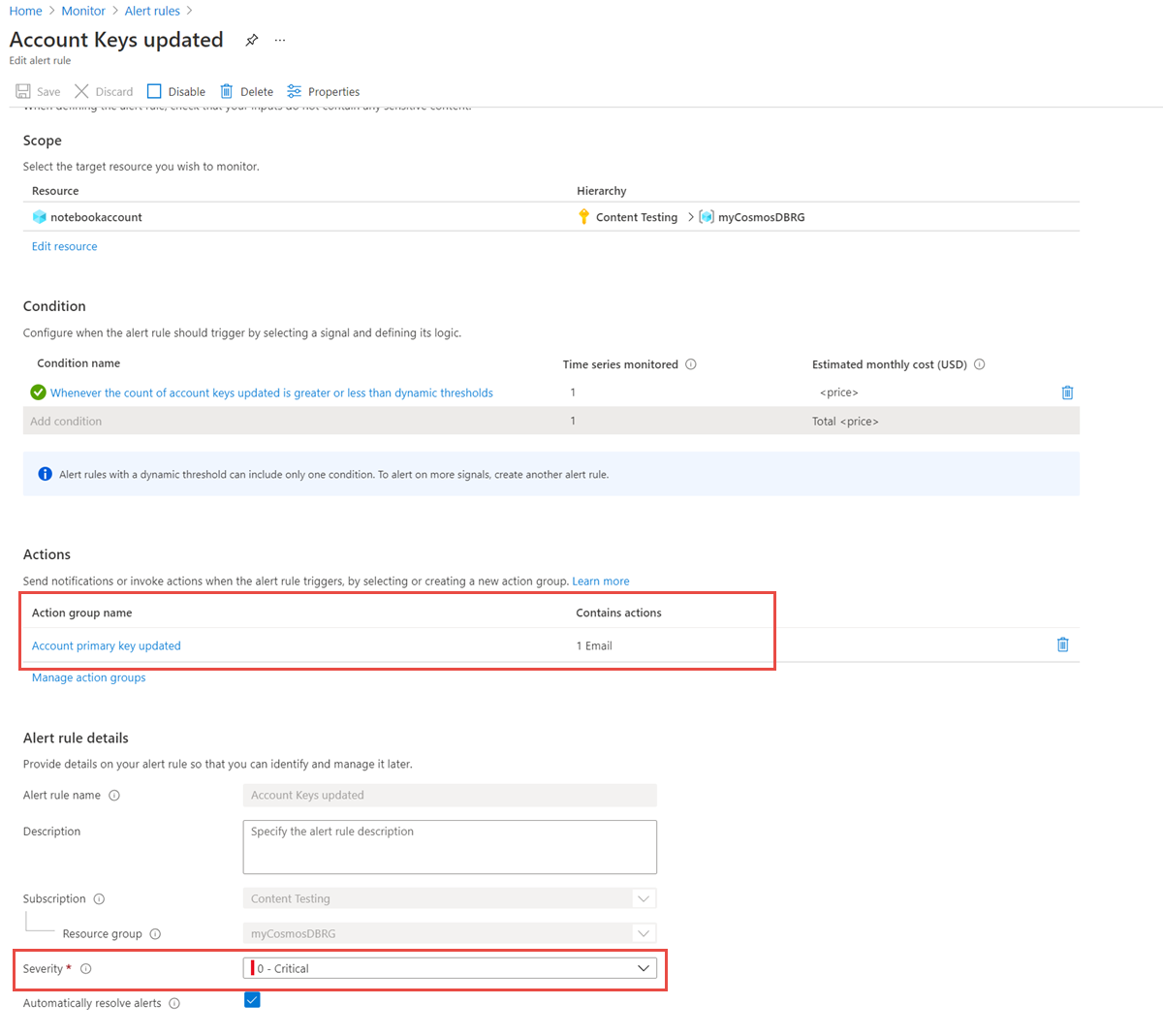**Detailed Caption for the Image:**

This page features a clean, white background, providing a crisp and clear view of the user interface elements. At the top left corner, the navigation path begins with the word "Home," followed by a right-pointing gray arrowhead. Next to "Home," the path continues with "Monitor" and another right-pointing arrowhead, followed by "Alert Rules" and yet another right-pointing arrowhead, indicating a breadcrumb trail of navigation. All these links are presented in a blue font.

Immediately below this navigation path, there is a prominent, bold black heading stating "Account Keys Updated." Positioned toward the right side of this heading, there is a gray pushpin icon, angled with its tip pointing to the lower left. Further to the right, three vertical dots are visible, suggesting additional options in a dropdown menu.

Beneath the main heading, the phrase "Edit Alerts Rule" appears in a light gray font, denoting a sub-section of the page. Following this, there are several actionable icons: a floppy disk icon labeled "Save," an 'X' icon labeled "Discard," and a blue-outlined checkbox labeled "Disable" with the word "Disable" in black. Additionally, there is a blue trashcan icon with the label "Delete" in black.

The page continues with a series of blue toggle buttons accompanied by the label "Properties." Below this section, a light gray divider line separates the content. Beyond the divider, the ends of a sentence are faintly visible but indiscernible.

Further down, in bold black text, the heading "Scope" is displayed. Underneath this, in non-bold gray text, the instruction reads, "Select the target resource you wish to monitor."

Another bold black heading, "Resource," appears next, followed by a sort of table. Within this table, the only listed option features a small, 3D blue box icon labeled "Notebook Account." Adjacent to this, a gold upward-pointing arrow accompanied by the text "Content Testing" with a right-pointing arrowhead in brackets is shown. Additionally, a smaller version of the 3D blue box icon appears with the label "my Cosmos DBRG," with "DBRG" capitalized.